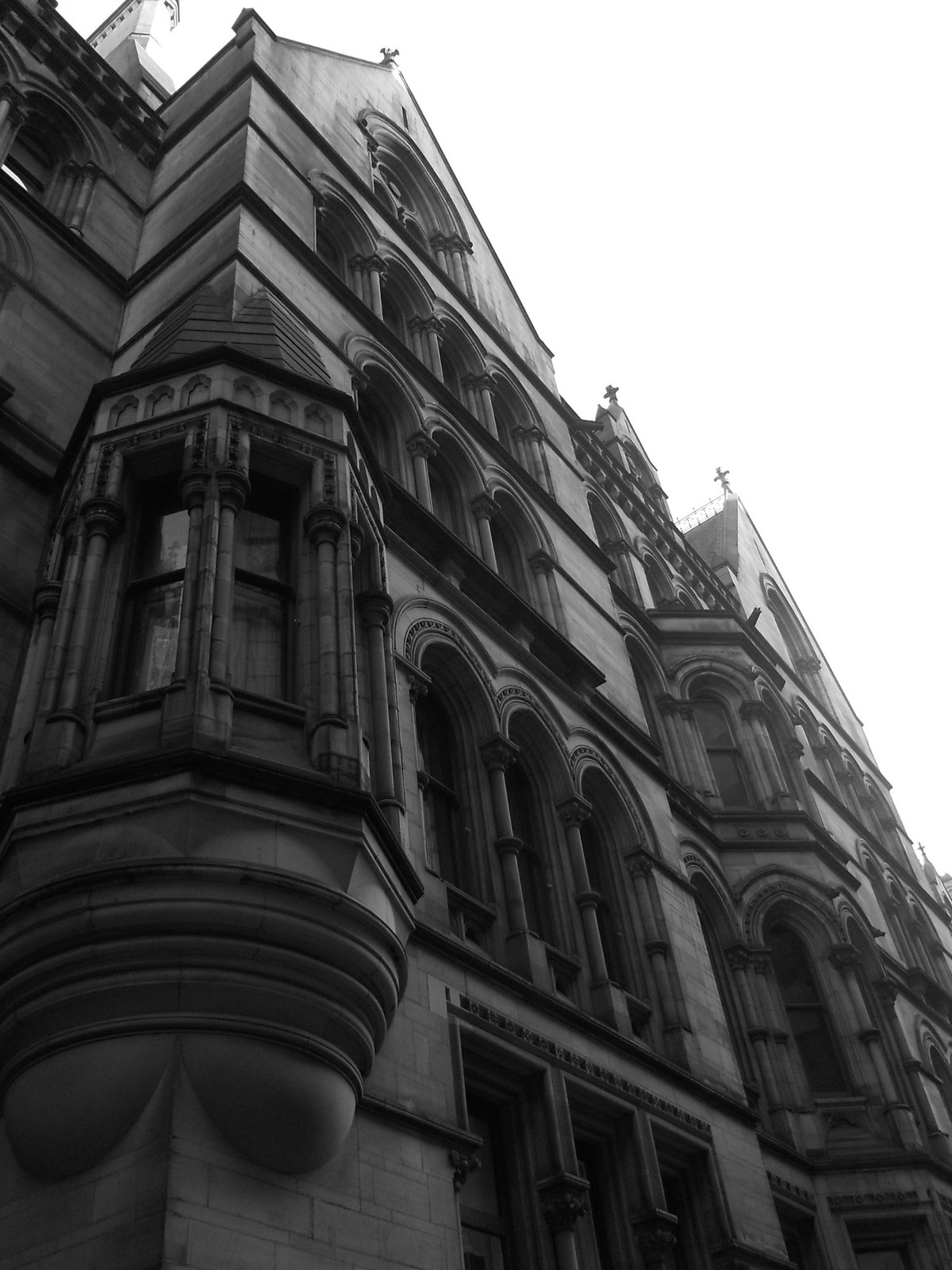This black-and-white photograph captures a tall, five-story building, likely a cathedral or church, in a European architectural style. Shot from a corner angle, the image looks upward from a sidewalk perspective, emphasizing the building's height and ornate details. The front facade features multiple rows of arched windows with decorative frames and rounded borders. The building is constructed from light-colored stone, adding to its grandeur. Various peaked roofs and gables accentuate the structure, each crowned with a spire or cross, indicating its religious significance. A distinctive window turret projects from the left side of the structure, adding a unique element to the architectural design. The photo’s dull sky, a result of the black-and-white medium, contrasts starkly with the intricate detailing of the building, highlighting its curves and gothic features. The perspective and the detailed, realistic style of the photography effectively convey the imposing and historic nature of the edifice.